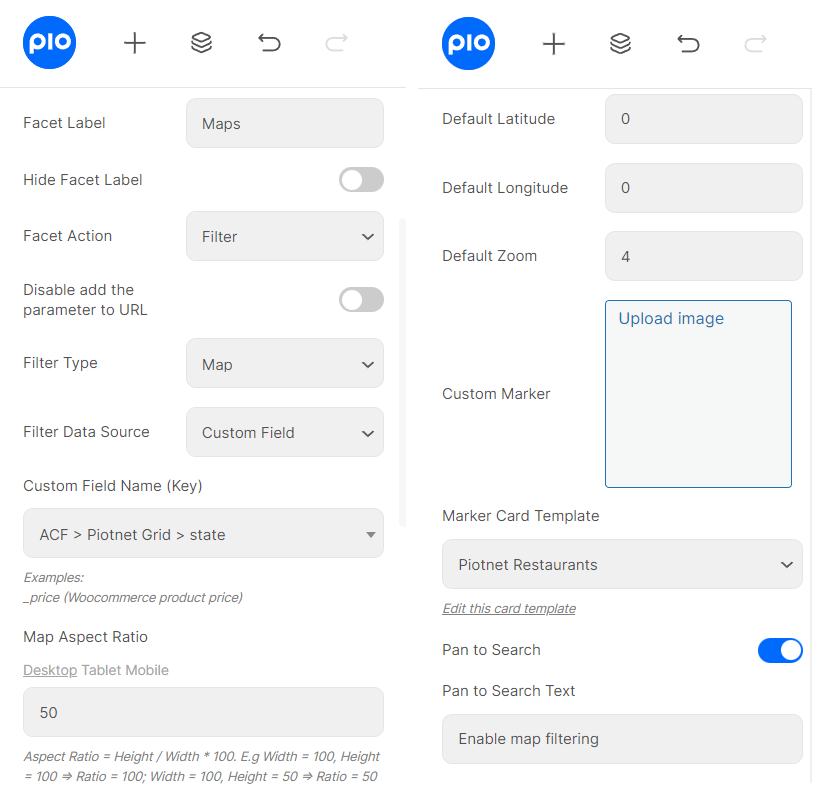This composite image showcases two screenshots of different settings pages for a mapping application, each replete with various customization options.

*In the first screenshot:*
- The interface prominently features a Pio icon in blue.
- Several icons are available, including a plus sign, a stack of squares, and a back arrow.
- Menu options are displayed, including "Facet Label" with sub-options such as "Maps" and "Hide Facet Label."
- The "Facet Action" is configured to "Filter."
- A toggle button for "Disable & Add Parameter to URL" is visible, currently turned off.
- Under "Filter Type," the selection is set to "Map," with "Custom Field" designated as the data source.
- The "Custom Field Name" specified is "ACF."
- Additional text includes "Pintant Grid" and "State," denoting changeable filters.
- The map's aspect ratio for desktop and tablet mode is set to 50, explained by the formula: Aspect Ratio = (Height / Width) x 100. Examples are provided: Width = 100, Height = 100, Ratio = 100; Width = 100, Height = 50, Ratio = 50.

*In the second screenshot:*
- The Pio icon remains consistent, featuring a blue background with white text.
- Labels indicate settings for "Default Latitude" and "Default Longitude," both set to zero.
- The "Default Zoom" level is established at 4.
- Options for a "Custom Marker" and a "Marker Card Template," set to "Pionte Restaurants," are available, with an option to edit the card template.
- The "Pan to Search" feature is enabled, with corresponding text stating "Enable Map Filtering."

Both screenshots feature a white background with gray text, resembling typical settings interfaces. Multiple customization settings are illustrated, enabling comprehensive control over map display and functionality.